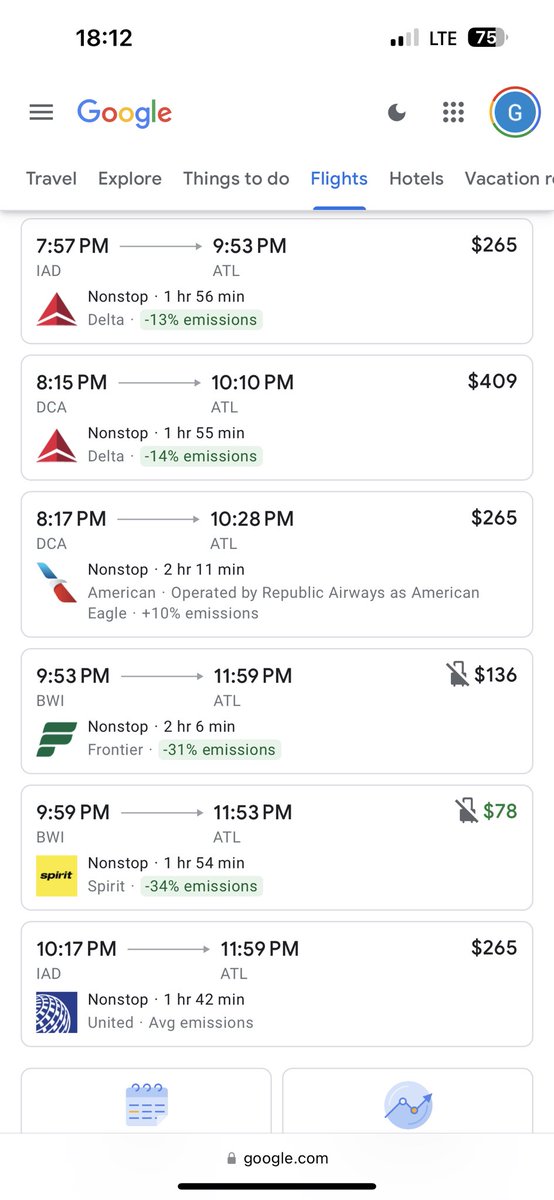A screenshot displaying a list of flight options from Washington D.C. area airports (IAD, DCA, BWI) to Atlanta (ATL). The detailed flight information is as follows:

1. **Flight 1:**
   - **Departure:** 7:57 PM from IAD
   - **Arrival:** 9:53 PM at ATL
   - **Duration:** 1 hour 56 minutes
   - **Airline:** Delta
   - **Price:** $265
   - **Emissions:** 13% below average

2. **Flight 2:**
   - **Departure:** 8:15 PM from DCA
   - **Arrival:** 10:10 PM at ATL
   - **Duration:** 1 hour 55 minutes
   - **Airline:** Delta
   - **Price:** $409
   - **Emissions:** 14% below average

3. **Flight 3:**
   - **Departure:** 8:17 PM from DCA
   - **Arrival:** 10:28 PM at ATL
   - **Duration:** 2 hours 11 minutes
   - **Airline:** American Eagle (operated by Republic Airways)
   - **Price:** $265
   - **Emissions:** 10% below average

4. **Flight 4:**
   - **Departure:** 9:53 PM from BWI
   - **Arrival:** 11:59 PM at ATL
   - **Duration:** 2 hours 6 minutes
   - **Airline:** Frontier
   - **Price:** $136
   - **Emissions:** 31% below average

5. **Flight 5:**
   - **Departure:** 9:59 PM from BWI
   - **Arrival:** 11:53 PM at ATL
   - **Duration:** 1 hour 54 minutes
   - **Airline:** Spirit Airlines
   - **Price:** $78
   - **Emissions:** 34% below average
   - **Note:** Includes a luggage icon with a line through it (likely indicating no checked luggage).

6. **Flight 6:**
   - **Departure:** 10:17 PM from IAD
   - **Arrival:** 11:59 PM at ATL
   - **Duration:** 1 hour 42 minutes
   - **Airline:** United Airlines
   - **Price:** $265
   - **Emissions:** Average

7. **Flight 7:**
   - **Departure:** 9:59 PM from BWI
   - **Arrival:** 11:59 PM at ATL
   - **Duration:** 2 hours
   - **Airline:** Frontier
   - **Price:** Not explicitly stated but inferred from the previous Frontier listing ($136).

Each flight listing includes details on departure and arrival times, flight duration, airlines, prices, and emissions relative to the average, providing a comprehensive comparison for travelers.